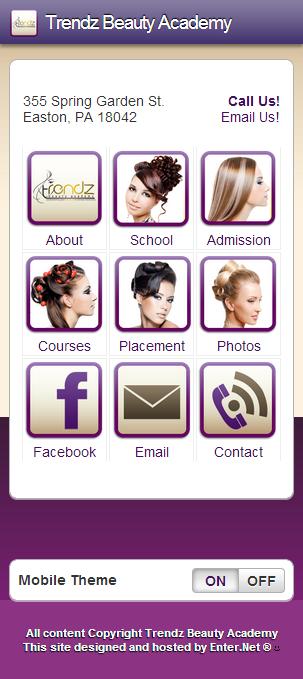The image showcases an advertisement for Trends Beauty Academy as viewed on a mobile device. At the top of the image, a blue-purple gradient banner displays the academy's name in white text: "Trends Beauty Academy" (with "Trends" spelled with a Z). Below, the screen resembles a phone interface, featuring a large white vertical rectangle that contains nine clickable squares. These squares, designed as rounded icons, link to various sections of the academy's website, including About, School, Admission, Courses, Placements, Photos, Facebook, Email, and Contact. The icons display either artistic drawings of women with varying hair colors or symbols such as the Facebook logo, an email envelope, and a phone emitting a Wi-Fi signal. The academy's address, 355 Spring Garden Street, Easton, Pennsylvania, 18042, is prominently displayed, along with contact prompts like "call us" and "email us." The bottom portion of the image features a predominantly purple background with a white text section that includes a mobile theme toggle (on/off) and a copyright notice: "All content copyright Trends Beauty Academy. This site designed and hosted by Enter.net." A small smiley face appears at the very bottom, adding a subtle, friendly touch.